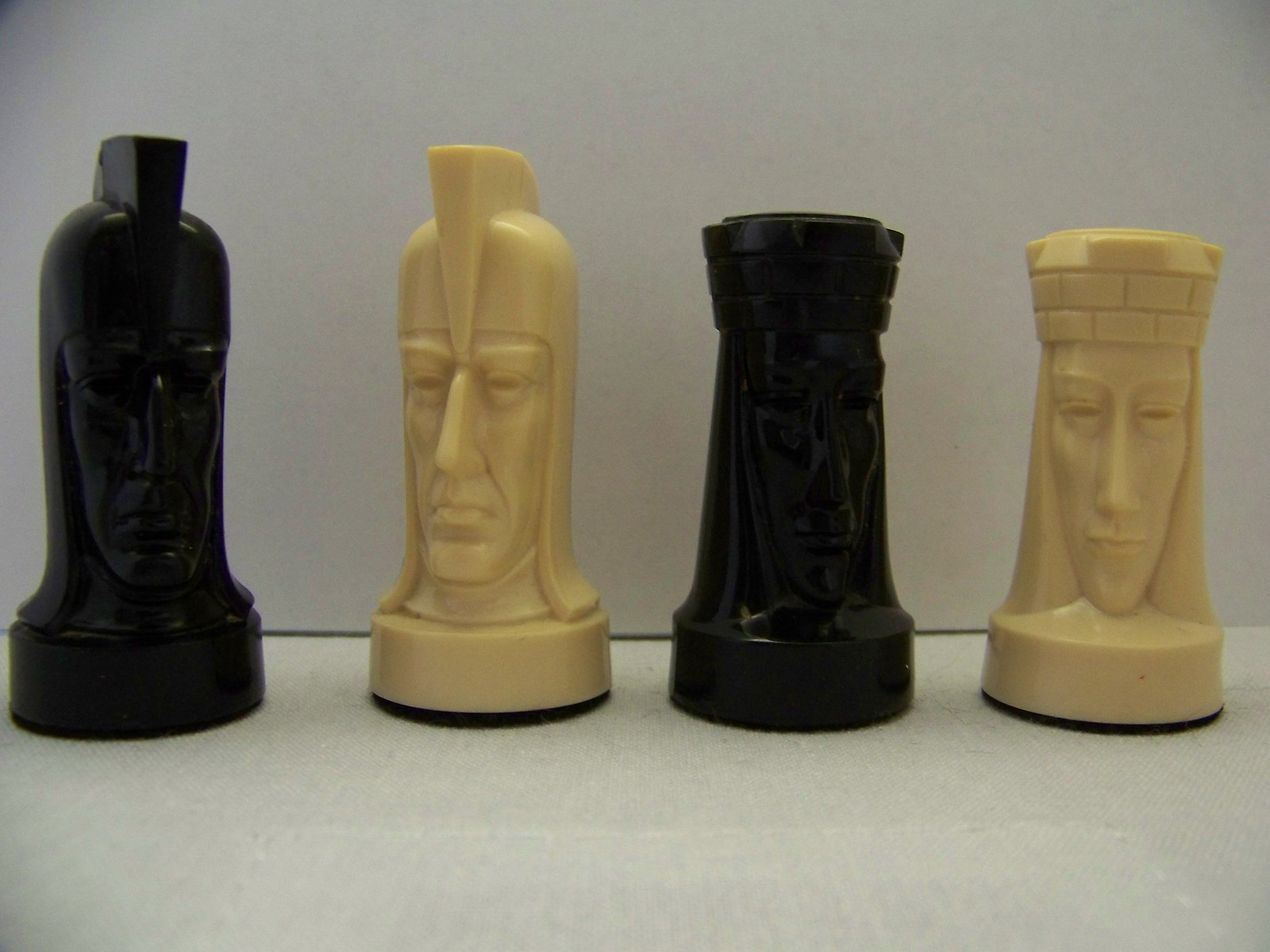The image displays four intricately carved figures resembling chess pieces, arranged on a subtly textured gray surface with a flat gray wall in the background. The pieces alternate in color, forming a black-beige-black-beige pattern. The two figures on the left appear to be male, each donning a helmet-like headpiece with a small ruffle or mohawk. These figures feature squared-off faces and pointed noses, suggesting a kingly or knightly appearance. The two figures on the right, colored black and beige respectively, are female, characterized by brick-like crowns and elongated faces rounded at the bottom, also with pointed noses and long hair. The detailed craftsmanship of the figures and their alternating pattern add a distinctive allure, suggesting their role as ornate game pieces or decorative chess elements.